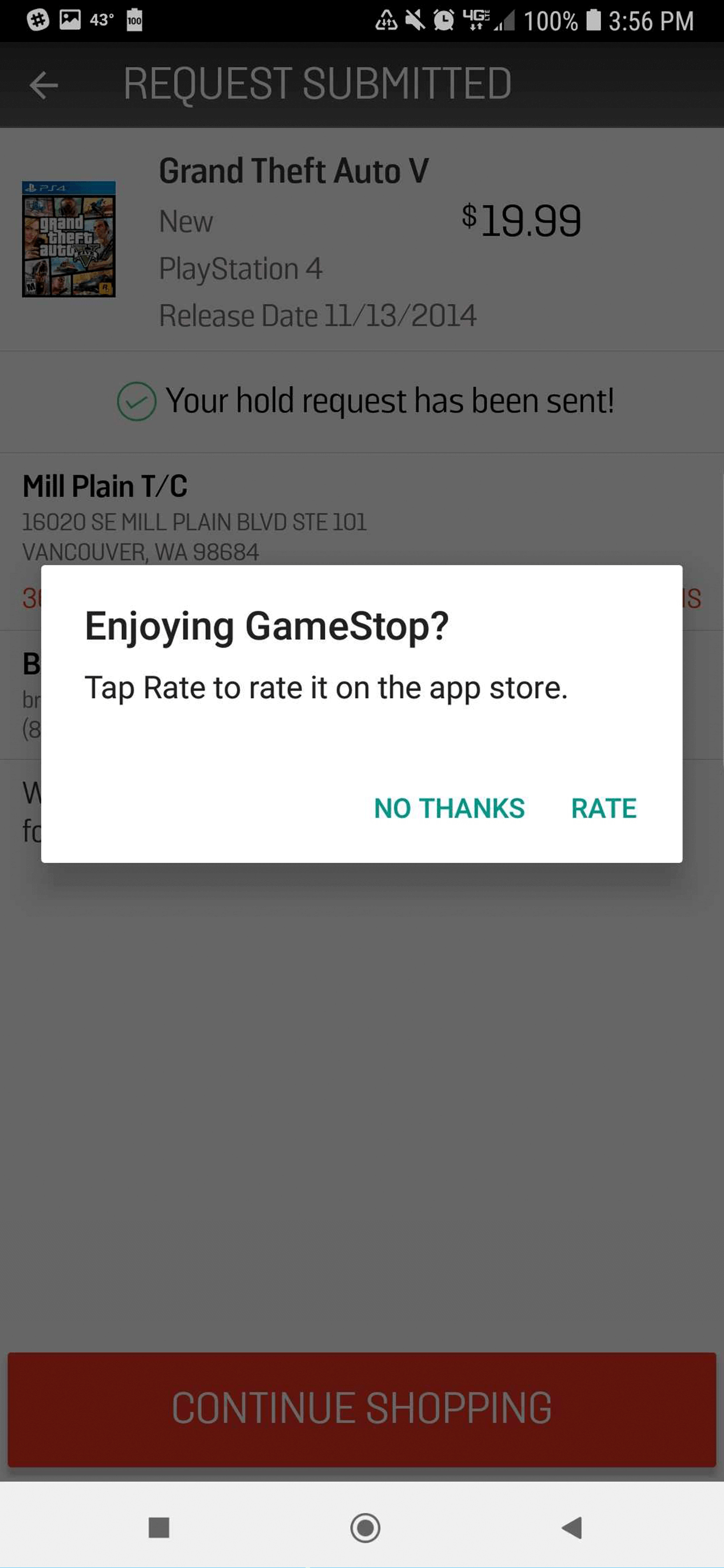This image appears to be a screenshot from a mobile phone, evidenced by its narrow, vertical rectangular shape. The top portion of the screenshot is dark, featuring various status icons against a black background. On the upper right, in white font, the time is displayed as "3:56 PM", next to a fully charged battery icon and "100%". Additional status icons can be seen on both sides of the top bar.

Beneath the top bar, a left arrow icon is displayed, followed by the text "REQUEST SUBMITTED" in all capital letters, though the text is somewhat muted and not fully visible. Below this, a smaller vertical rectangular image shows the game's cover, “Grand Theft Auto”, with the title “Grand Theft Auto 5” printed to the right of the image in black font. On the left of this section, "NEW" is displayed, followed by the price "$19.99" in bold font. Below "NEW", it specifies "PlayStation 4" and mentions the release date as "11-13-2014". 

Further down, a green circle with a checkmark inside it signifies confirmation, accompanied by the bold text "Your hold request has been sent." The next section lists the address for "Mill Plain T/C" in black bold font but is overlaid by a white pop-up message that asks, "Enjoying GameStop?" in bold, and urges users to "Tap rate to rate it on the App Store". At the bottom right of this pop-up are two green options: "NO THANKS" and "RATE," both in capital letters.

Towards the very bottom, an orange rectangular horizontal button displays "CONTINUE SHOPPING" in white capital letters. At the very bottom in a white area, several icons are faintly visible, including a filled square, a circle with a dot inside, and a left arrow.